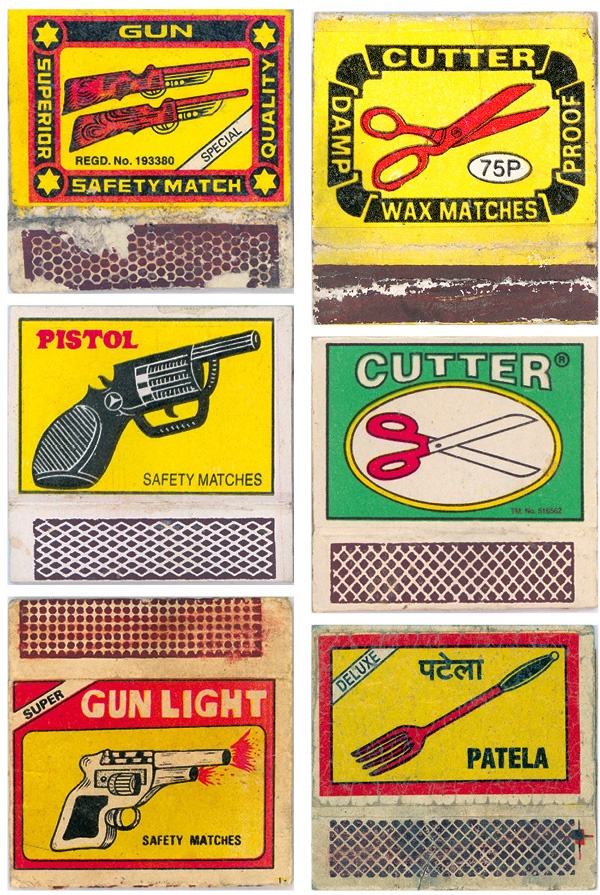This photo features six antique matchboxes, each uniquely designed and showcasing intricate vintage illustrations. Arranged in three vertical columns, the boxes are all square in shape and exhibit a captivating array of imagery and text.

**Left Column:**
1. **Top Box:** Displays two red guns set against a yellow background bordered in black. The text reads, "Safety Match, Quality Superior."
2. **Middle Box:** Features a black pistol with the label "Pistol Safety Matches."
3. **Bottom Box:** Showcases another pistol, marked as "Super Gun Light Safety Matches."

**Middle Column:**
1. **Top Box:** Contains imagery of red scissors, against a yellow background with the text "Wax Matches" and "Damp Proof." The price "75 pence" is also visible.
2. **Middle Box:** Presents a large pair of scissors with "Cutter" written in white text, contrasting on a green background.
3. **Bottom Box:** Highlights a long fork with the labels "Deluxe Patella," written both in English and Hindi, on a yellow background accented with red.

**Right Column:**
1. **Top Box:** Includes a smaller pair of scissors with a red handle and white text "Cutter" on a green background.
2. **Middle Box:** Another scissor design, with text indicating "Wax Matches," and a red handle.

Each matchbox bears a distinct pattern on its striking surface, ranging from solid and crisscross to circular designs, some of which show signs of past use, adding to their nostalgic allure. The majority of the matchboxes feature a predominant yellow hue, with the exception of one box in the middle right, which breaks the pattern with a green background. These vintage collectibles, likely from the 1930s or 1940s, evoke a bygone era and are a testament to the rich history of matchbox art.